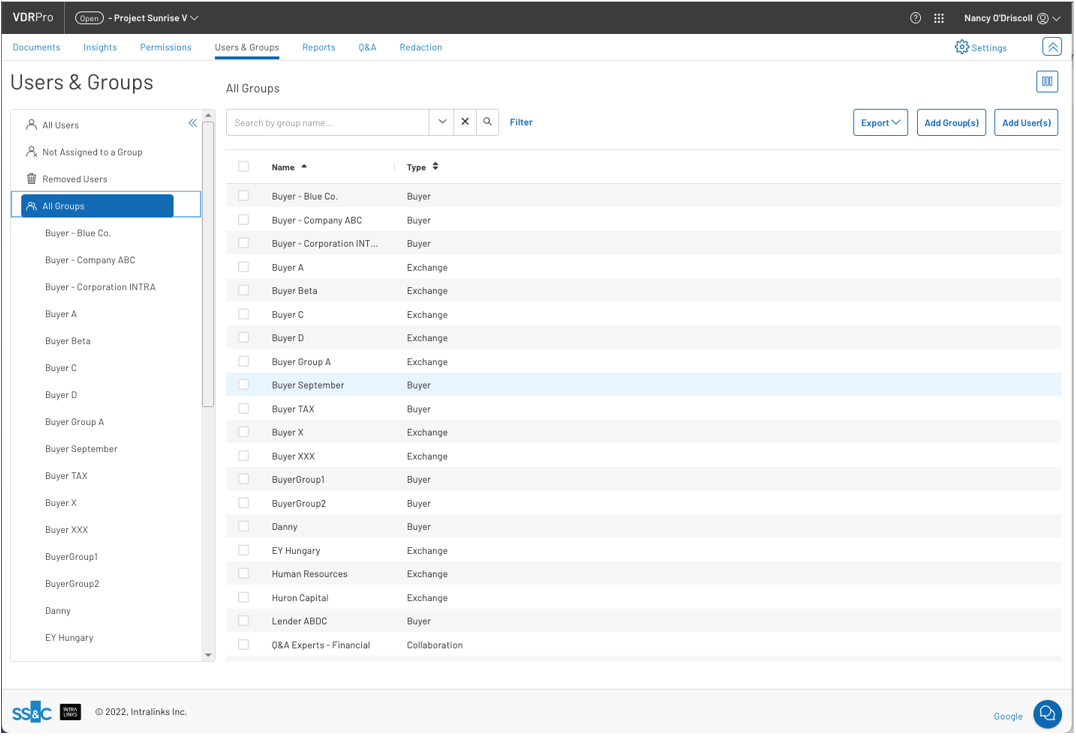The webpage displayed appears to belong to a platform named VDR Pro. At the top, it features an open project titled "Project Surprise and Ruminomeral V." On the right side, the screen indicates the account owner, Nancy O'Driscoll. The interface is divided into two main sections:

On the left section, there's a series of options under the "Users and Groups" category: 
- A list of All Users Not Assigned to a Group
- Removed Users
- A detailed listing of All Groups

The right section provides detailed listings of these groups, with columns for Name and Type. For instance:
- The first group is "Buyer Blue Company" categorized under the type "Buyer".
- Multiple other groups follow, categorized under different types such as Buyer and Exchange, in a specific order: Three Buyers, six Exchanges, two Buyers, two Exchanges, three Buyers, three Exchanges, and one Collaboration.

Additionally, the webpage offers other navigation features, including:
- Documents
- Insights
- Permissions
- Users and Groups
- Reports
- Q&A
- Reflection

At the bottom of the page, there is a chat feature for user interaction.